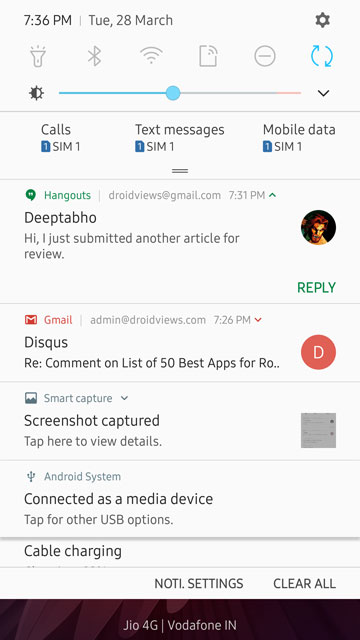In this image, we see a fully pulled-down notification bar from a smartphone. The wallpaper is barely visible at the bottom of the screen, partially displaying the text "Vodafone IN," indicating the location is India. At the top, the status bar shows the time as 7:36 p.m. on the 28th of March. Various icons from applications appear on the screen. The first notification is from Google Hangouts, with a message from a person named Deep Tabho that reads, "Hi, I just submitted another article for review." Below that, there is a Gmail notification from Disqus (spelled D-I-S-Q-U-S) about a reply to a comment on a list of the 50 best apps. Further down, there is a notification indicating that a screenshot has been captured. Finally, the Android system notification informs the user that the device is connected as a media device and prompts them to tap for other USB options.